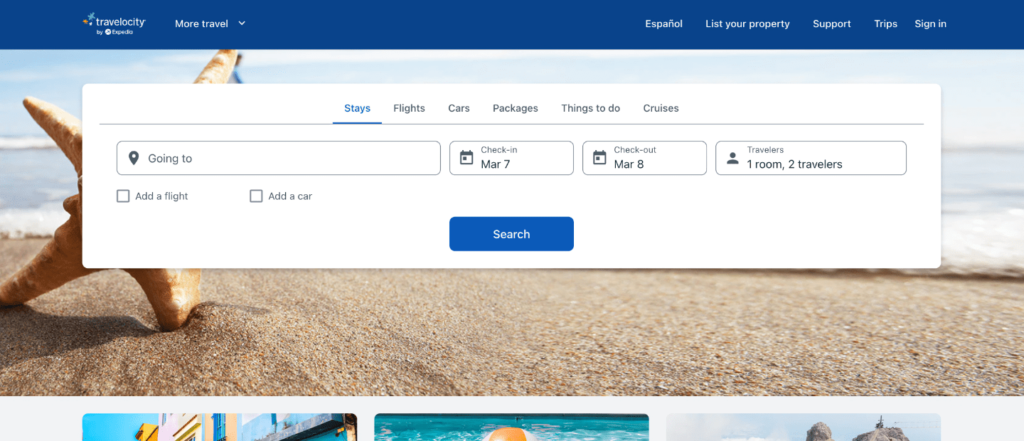This screenshot captures the top section of the Travelocity website. Dominating the top is a dark blue banner. In the top left corner, the "Travelocity" logo is prominently displayed, although the two words beneath it are difficult to discern due to the small size of the screenshot. Immediately to the right of the logo, there's a clickable text that reads "More to Travel," accompanied by a downward arrow, indicating a drop-down menu.

On the right side of the banner, a series of navigation options are available in white text: "Español," "List your property," "Support," "Trips," and "Sign in." Below this banner, the key search functionalities of the site are arranged in a user-friendly layout.

Centered on the page, a set of search options is offered through various tabs: "Stays," "Flights," "Cars," "Packages," "Things to Do," and "Cruises," with the "Stays" tab highlighted in blue. Directly beneath this tab, users can input their destination in a text box labeled "Going to." To the right, dropdown boxes allow users to specify their check-in and check-out dates, here shown as March 7th and March 8th, respectively. Further to the right, another dropdown box, labeled “Travelers,” displays "One Room, Two Travelers."

Additional search enhancements are available below the destination text box. Two checkboxes allow users to add a flight or a car to their booking search. Completing this section, a prominent blue search button with white text is centrally located at the bottom of these search options.

The background features a serene beach scene, including sand, gentle waves, and what appears to be either a shell or a starfish nestled in the sand. At the bottom of the screenshot, partial images of additional webpage tiles are visible but cut off, indicating more content below.